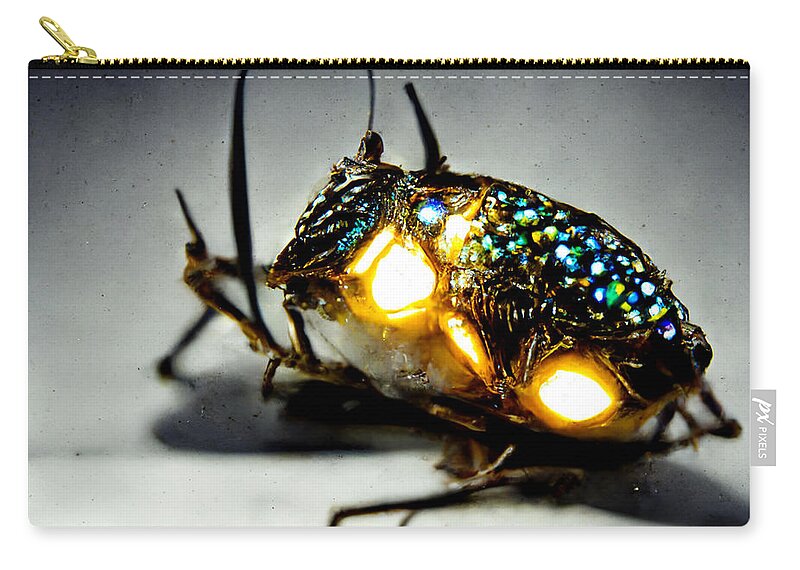This is a meticulously edited product photograph suitable for commercial use, featuring a zipper bag placed against a flat white background. The bag is adorned with a bronze gold-colored zipper at the top, with the tab positioned on the left side. Along the right edge, there is a gray banner that reads "PX pixels." Showcased prominently on the bag is a fantasy-themed beetle with two glowing yellow eyes and antennae, perched on intricate, slender, thorned branches. The back of the beetle is elaborately decorated with an array of blue and green gems, and it radiates three luminous dots, giving it an ethereal, neon-light effect. The beetle appears simultaneously realistic and like a jeweled brooch, with detailed legs and a textured body crafted to capture light, adding to its whimsical appeal. Despite the high level of detail, the image of the beetle appears digitally superimposed rather than printed directly onto the material of the zipper bag.